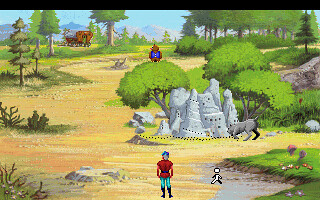The digital artwork depicts a meticulously crafted outdoor forest scene reminiscent of a 1990s point-and-click adventure game in pixel art style. Central and foreground is a character with their back facing the viewer, dressed in blue tights, black knee-high boots, and a red short-sleeved shirt, standing on a brownish-yellow dirt path. Adjacent to the character is a small white and black stick-figure-like shape with a circular head. In front of them is a small stone structure resembling a tiny castle adorned with white dot-like windows. A gray dog is seen sniffing the right side of this stone formation, adding an endearing touch to the scene. Behind the structure, a green-leaved tree stands tall with a brown owl perched atop. To the right, two additional trees frame the scene, while a brown wagon or carriage is faintly visible in the background, making its way into the distance. The backdrop is completed with a blue sky, verdant mountains, and a trio of trees flanking the view, encapsulating the essence of a tranquil, pixelated adventure world.